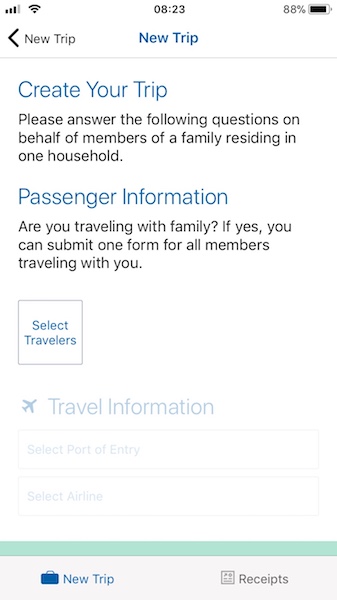The image depicts a user interface on a white background, designed for inputting travel information. Central to the image is a prominent title in blue saying "Create Your Trip," accompanied by the number "823" and the phrase "new trip" displayed twice. Below the title, there is a bold blue indicator showing "88 percent," possibly an indication of progress or confirmation.

The interface prompts the user to answer questions on behalf of family members residing in one household, asking specifically for passenger information. It includes the question, "Are you traveling with family?" with the note that if so, travelers can submit one form for all members. Further down, users are instructed to select travelers, provide their travel information, choose a port of entry, and select an airline.

On the right side, there is a noticeable green rectangle, possibly a button for further interaction. Above the green rectangle is a gray bar, serving as a divider or progress indicator. At the bottom of the interface, there are icons depicting a blue suitcase labeled "new trip" and a gray receipt, which is labeled "receipts" and shows an image of a traditional paper receipt.